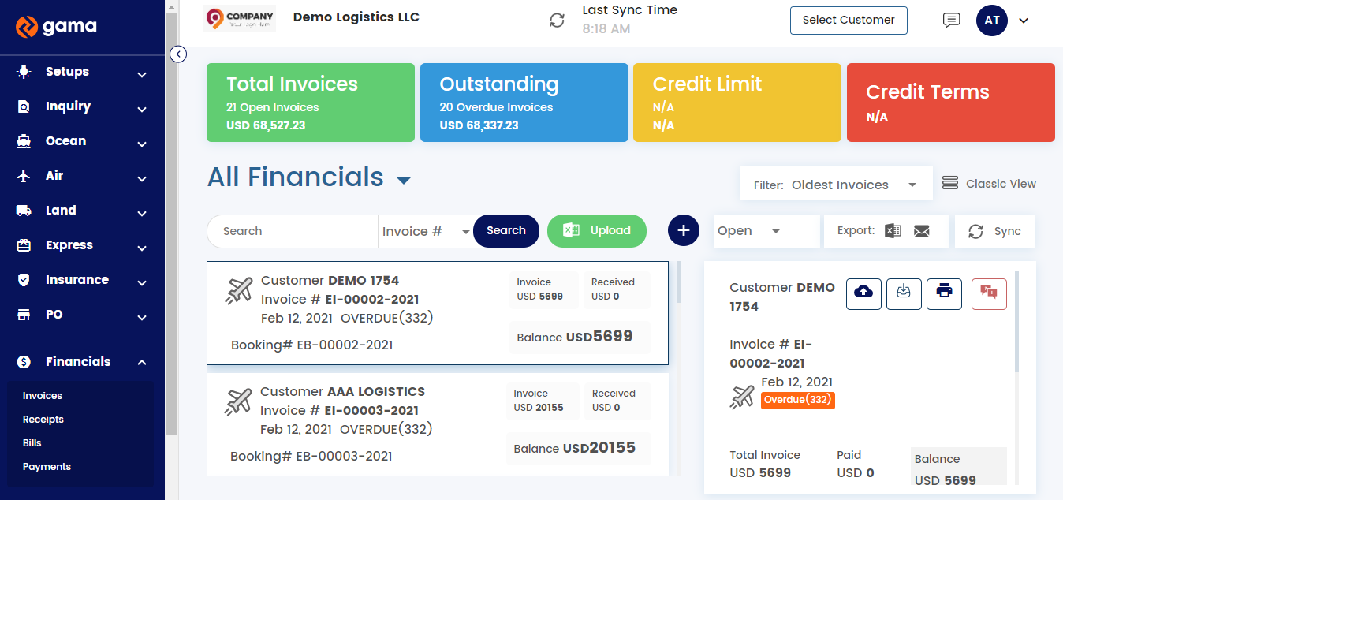A screenshot of a digital interface, possibly from a website or app named "Gamma," showcases its organized layout. On the left side, there is a vertical blue column featuring the "Gamma" logo at the top, accompanied by navigation menu options in white font. These options include "Setups," "Inquiry," "Ocean Air," "Land Express," "Insurance," "PO," and a subsection under "Financials" that lists "Payments" and "Bills."

In the main content area, the top row displays the title "Company Demo Logistics LLC," along with information about "lost sync time" and a button labeled "Select Customer." At the far right end of this row is a black profile button with the initials "AT."

Below the top row, four large and vividly colored buttons (green, blue, yellow, and red) span horizontally across the screen. These buttons provide detailed metrics about "Total Invoices," "Outstanding Invoices," with specifications in USD, "Credit Limit," and "Credit Terms."

Further down, there are additional informative sections. One section highlights invoice information, noting categories like overdue invoices. Other elements include a "Customer Demo" box, a search function, and an upload option. This lower part of the interface is predominantly white, supplemented by brightly colored buttons in shades of purple and green, contributing to a clean and informative user experience.